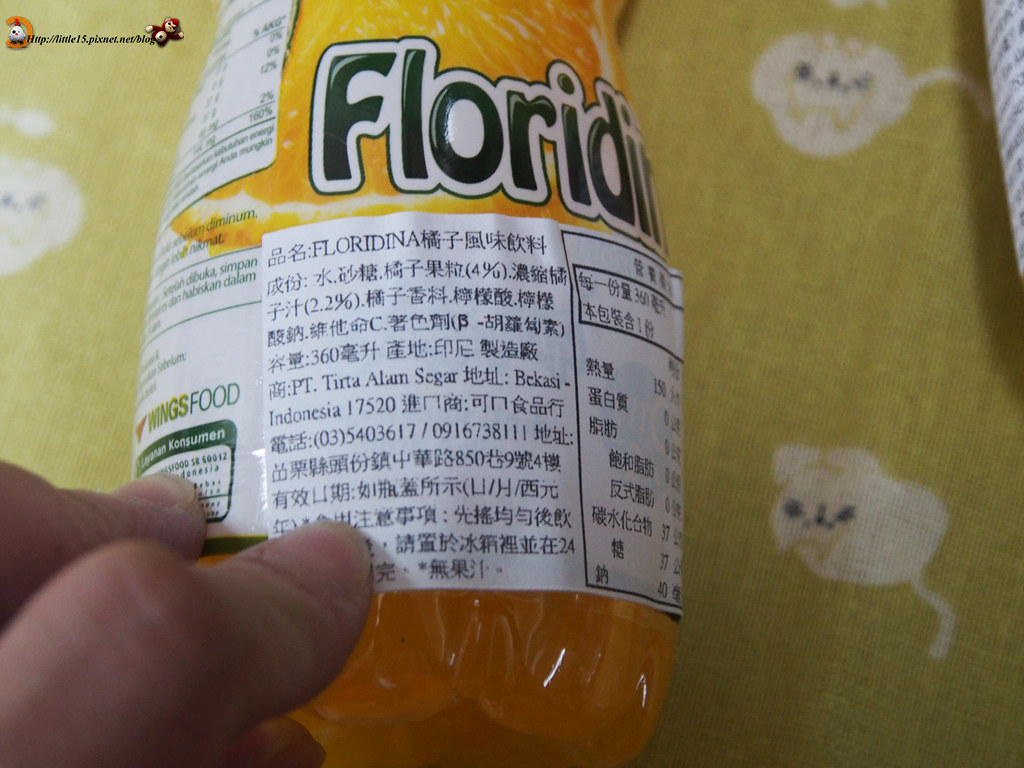The image features a cute green background adorned with multiple white animals, which appear to be either cats or dogs. On the bottom left-hand side, a pair of fingers is holding down a bottle filled with an orange fluid. The bottle's label states "Floridina" in green lettering on a white background. Notably, the nutritional facts on the label are written in Chinese characters. Additionally, there's a URL on the upper left-hand side displaying small icons of a chicken and a monkey, though the URL text itself is unclear.